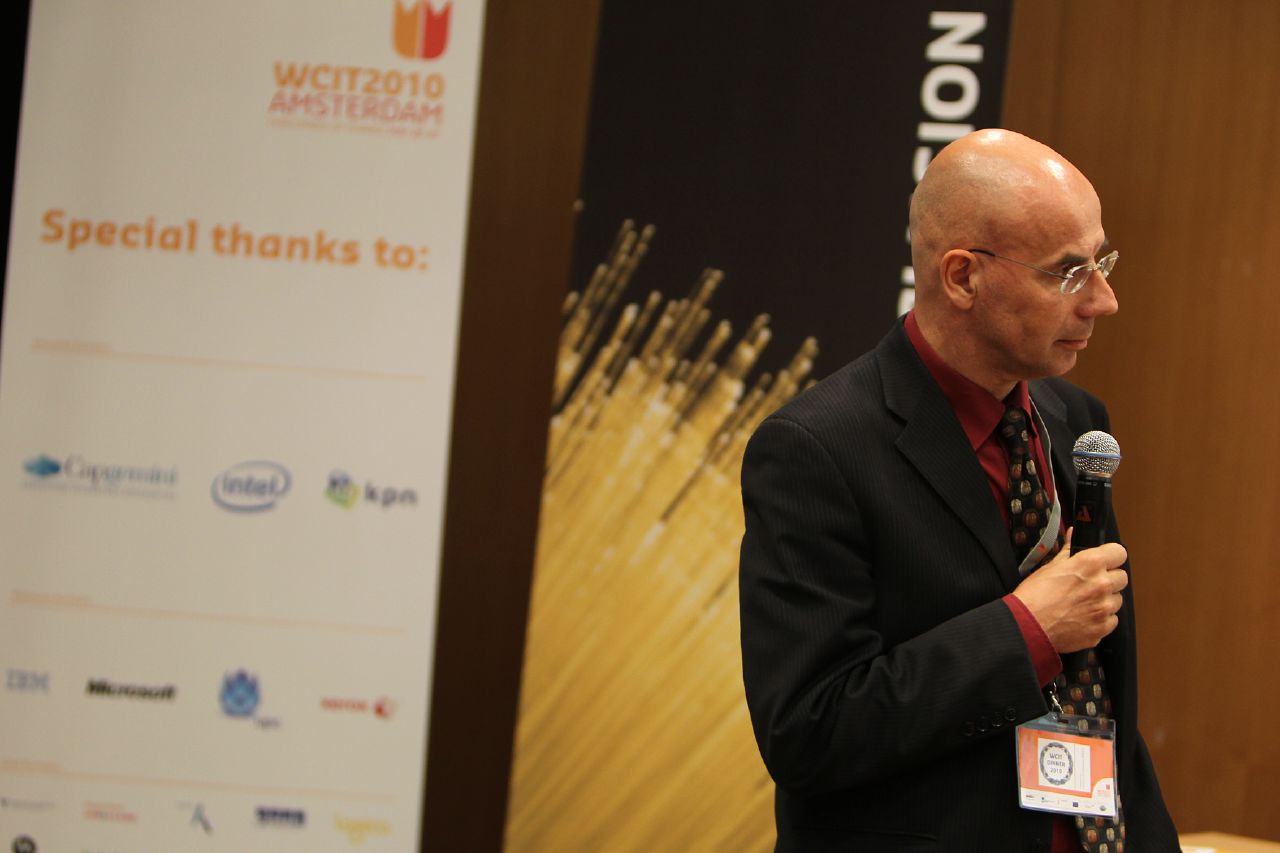This indoor photograph is rectangular, wider than it is tall, featuring a detailed scene predominantly in the right half of the frame. On the left-hand side, there's a white banner with an orange and red divided crown at the top, bearing the text "WCIT 2010 Amsterdam." Below this, in orange, it reads "Special thanks to," listing sponsors such as Intel, IBM, and Microsoft, though some logos remain indistinct. Adjacent to this is a brown wood-grain wall, followed by a black banner with yellow strands resembling wheat or fiber optic lights in the lower left-hand corner. The banner displays the letters "ION" vertically in white text on the right.

In the forefront stands a bald man, seen from the waist up and looking to the right. He has clear, circular glasses with white frames and is holding a microphone in his right hand. The man is dressed in a black suit jacket over a burgundy collared shirt, paired with a multi-colored tie featuring black, burgundy, and gold squares. Around his neck, he wears a laminated name tag on a red lanyard emblazoned with a small circle containing text. The backdrop and his poised demeanor suggest he is likely addressing the audience or about to speak at the event.